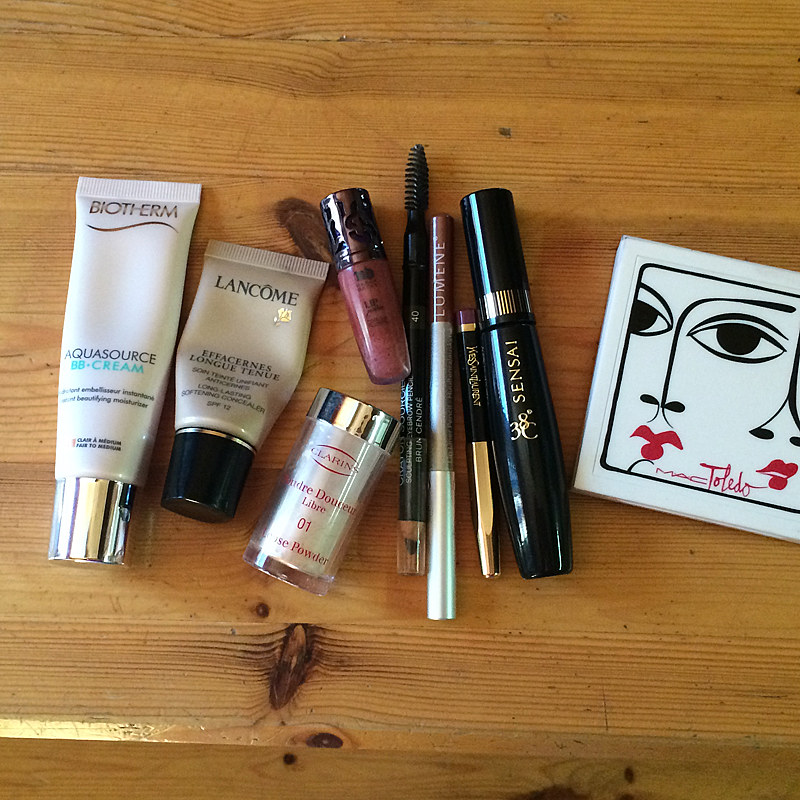The photograph showcases a neatly arranged collection of daily makeup essentials resting on a light yellow pine table. The collection includes an assortment of small jars, tubes, and pens. Two small jars can be seen, one possibly containing lipstick and the other holding a type of powder. There's also a Biotherm Aquasource cream and a Lancome tube, presumably containing makeup. Additionally, two types of lotion are visible, both in small containers. Four makeup pens are prominently displayed, marked as Lumine and Sensai, among others, likely for eyeliner and mascara. A card or printed material with a design featuring two eyes, lips, and the word "Toledo" adds a touch of artistic flair to the setup. The overall scene is meticulously organized, emphasizing the variety and detail of the makeup collection.